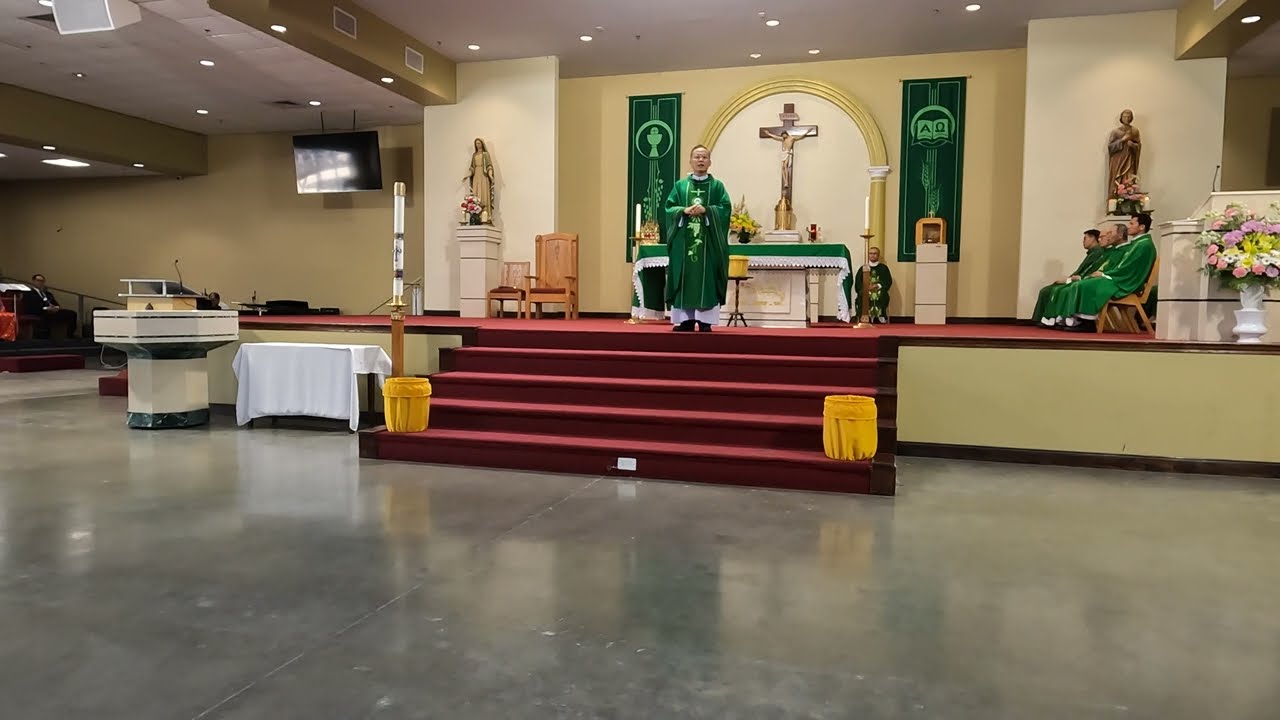The image depicts a grand church interior, characterized by its large, rectangular space that is about twice as wide as it is tall. Dominating the scene is an altar elevated on a stage-like platform, accessible by five wide stairs covered in a lush dark red carpet. The carpet extends up to the altar, which is set against a backdrop of recessed beige walls featuring scattered circular lights and a central, lighter brown or pale gold recess.

In the center of the altar stands a priest or minister dressed in a deep green robe, flanked by four other priests or ministers seated to his right, also donned in matching green attire. Beneath the main robe, the standing priest's white pants and black shoes are visible. Behind the altar, a crucifix is prominently displayed within a gold, arched framework, adding an element of reverence. Flanking the arch are two green banners, in harmony with the priests' robes.

To the left of the altar, a statue of Mary stands on a pedestal, while another statue, potentially of Jesus, is more faintly visible on the far left of the stage, both contributing to the solemn atmosphere. Adding to the décor are large arrangements of pink and yellow flowers in a white vase positioned at the right edge of the stage. The platform itself is fronted by a low yellow wall, contrasting with the red carpeted steps.

On the first step, several gold, cloth-covered containers that resemble buckets or trash cans can be seen, adding an intriguing element to the scene. The area beneath the altar table is also green, matching the dominant color theme. The shiny floor in the lower half of the image, possibly made of tile or stone, reflects the altar and those present, enhancing the overall luminance and grandeur of the setting.